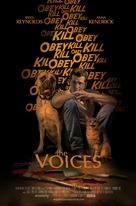The poster for the film "The Voices" features a small, VHS cassette-esque advertisement centered around a white man seated on a brown floor against a black backdrop. The man, dressed in blue jeans and a white polo shirt, sits with his knees up and his arms resting on them, hands clasped together. He is flanked by a large dog, possibly a boxer, on his right, and in front of him lies an orange cat with a creepy smile. Scattered around the man are various items that appear to be murder weapons, hinting at a violent theme. Above him, in a variety of sizes, the words "Kill" and "Obey" are repeated in gold font. Additionally, actor names are listed in the top left corner with production credits dispersed across the top right and bottom of the poster. Below the seated man, the film's title, "The Voices," is prominently displayed.